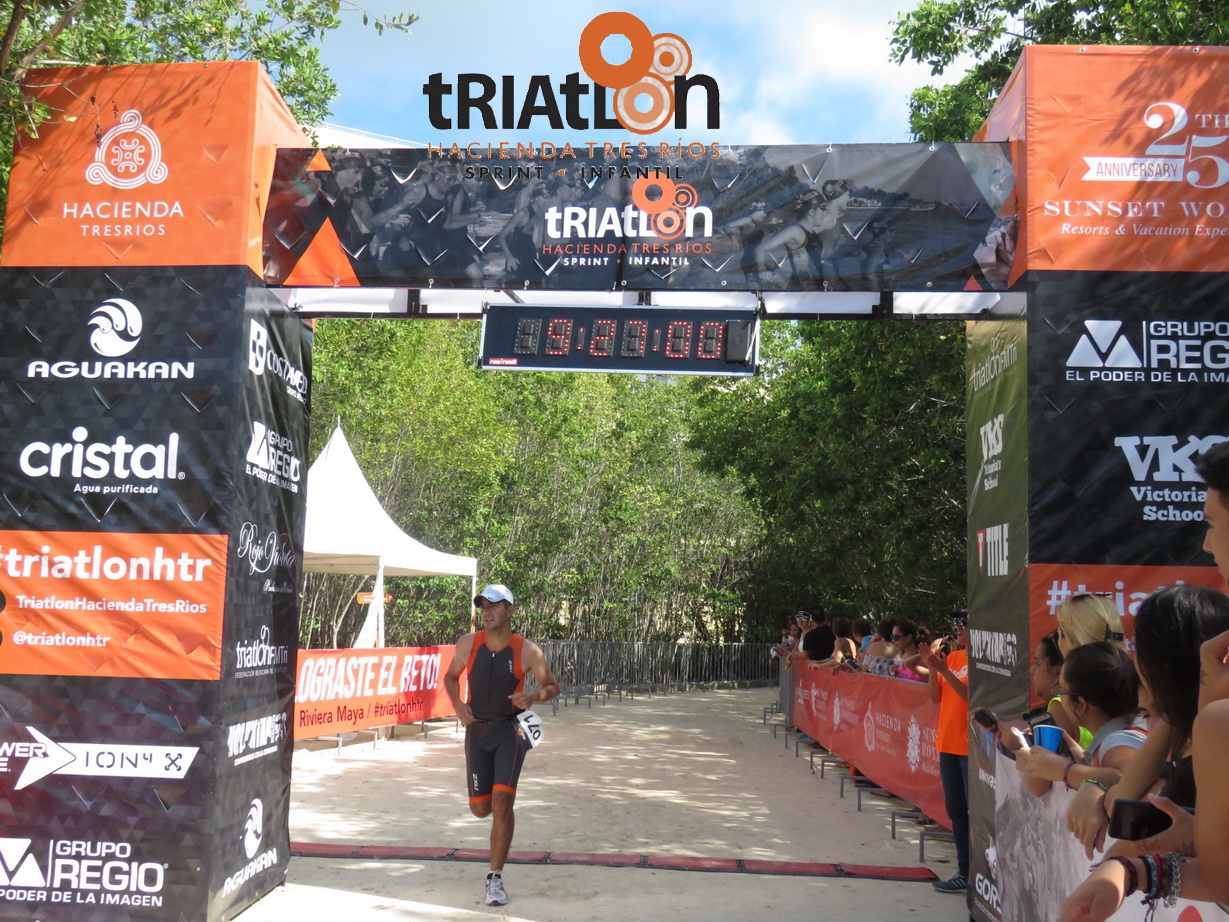The image captures the vibrant finish line of a triathlon on a sunny day. An archway constructed from scaffolding and covered with printed vinyl banners dominates the scene. The banners feature numerous sponsor logos, including Hacienda Tresorios, Aquacon, Crystal, Webion IX, Group Reggio, VK Victoria School, and Sunset 2.5. The word "Triathlon" is prominently displayed at the top in white letters on a black background, accented with orange highlights. Beneath it, "Hacienda Tresorios" and "Sprint Infantile" are printed in orange and white.

An LED clock above the archway shows a time of either 9:27 or 5:27, suggesting a lengthy race duration. A runner in his early 40s, clad in black spandex with orange embellishments, crosses the finish line. The dirt pathway he's running on is lined with cheering spectators who are kept back by gated barricades. To the left, a white canopy with an orange banner below it, complements the scene, while trees in the background frame the energetic atmosphere.